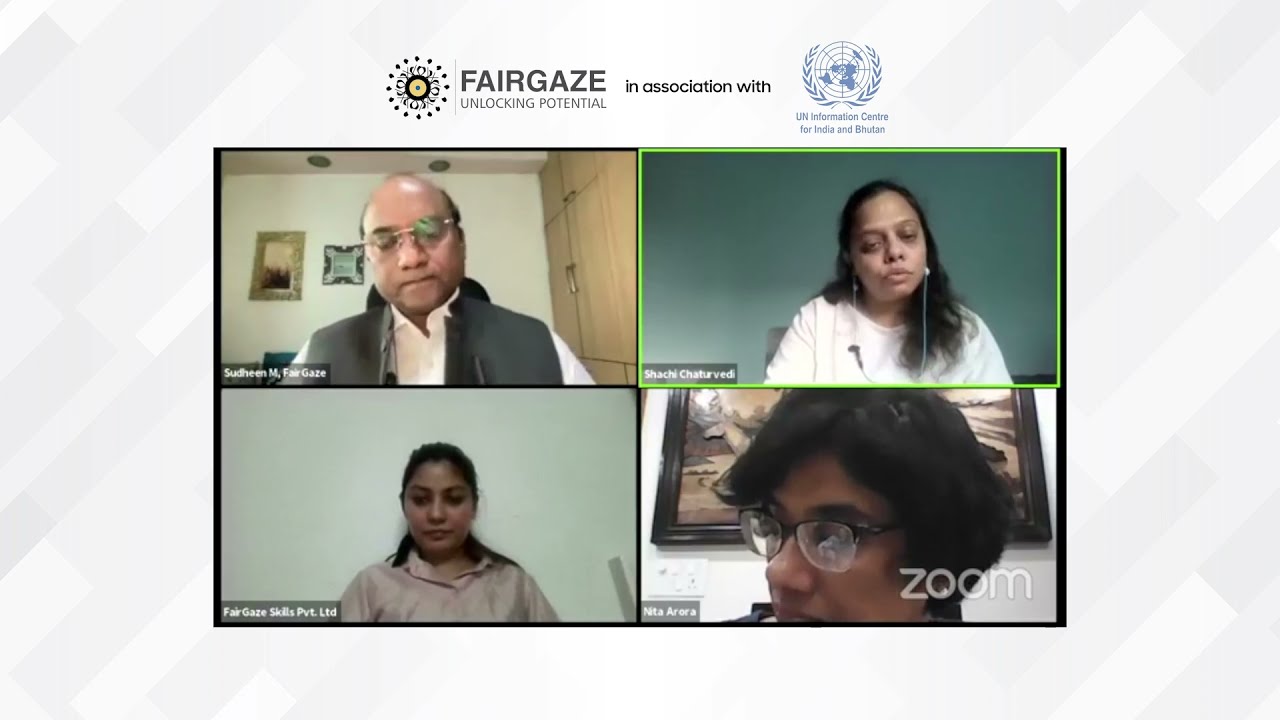The detailed image is a color screenshot of a Zoom meeting inset into a white background slide. At the top of this white area, there is the title "FAIRGAZE" with the subtitle "Unlocking Potential." To the left of this text, there is a circular logo with a spiral design. On the right, there is a blue-colored logo resembling the United Nations symbol, specifically denoted as the "UN Information Center for India and Bhutan."

The Zoom meeting screen itself is divided into four equally sized panels, with each panel displaying a different participant. In the top left, there is a balding man with glasses, wearing a white shirt and a gray vest, possibly named Sudevan. The top right displays a woman in a white sweater and earphones, appearing to be in her 50s with eyes partly closed, indicating she might be the active speaker since her frame is outlined with a green border. In the bottom left, there is another woman with long dark hair, wearing a pink shirt. The bottom right features a person with short black hair and eyeglasses. All participants appear to be of Indian descent.

Additionally, the Zoom logo is present in the bottom right corner of the meeting screen. The entire screenshot is set against a patterned background with gray and white diagonal planking, creating a Photographic Representationalism Freeze Frame Video style. The mood captured suggests a formal or professional meeting rather than a casual family call, as inferred by the serious expressions on the participants' faces.